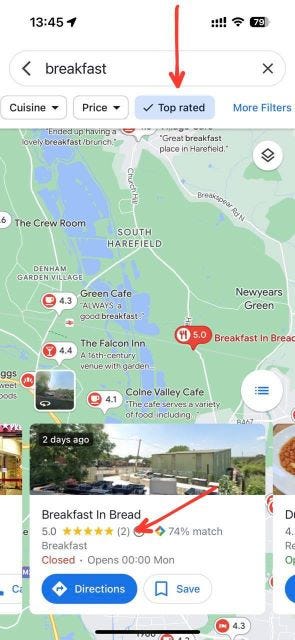The image displays a screenshot from a smartphone. At the top, the screen's white border frames the status bar. On the left side of the bar, the time is shown as 13:45. On the right side, the battery icon indicates a charge level of 79%. The screenshot appears to be from a Google interface, perhaps Google Maps or a Google search page. At the top, the search query "breakfast" is entered. 

Below the search bar, four filter options are available: Cuisine, Price, Top Rated, and More Filters. The "Top Rated" filter is selected, highlighted in blue with a checkmark beside it. A red arrow is drawn pointing to this selected filter.

Further down, a portion of a map is visible, though the city is not identifiable. A green area, possibly a park, is labeled "South Harefield." Several location markers with labels are visible, including "Green Cafe," "The Falcon Inn," "Cone Valley Cafe," and "The Crew Room." 

At the bottom of the screen, a photograph of a restaurant listing named "Breakfast in Bed" is visible. The establishment has a five-star rating but only two reviews. An arrow points to this listing. Below the restaurant's details, a blue button with rounded edges and white text reads "Directions."